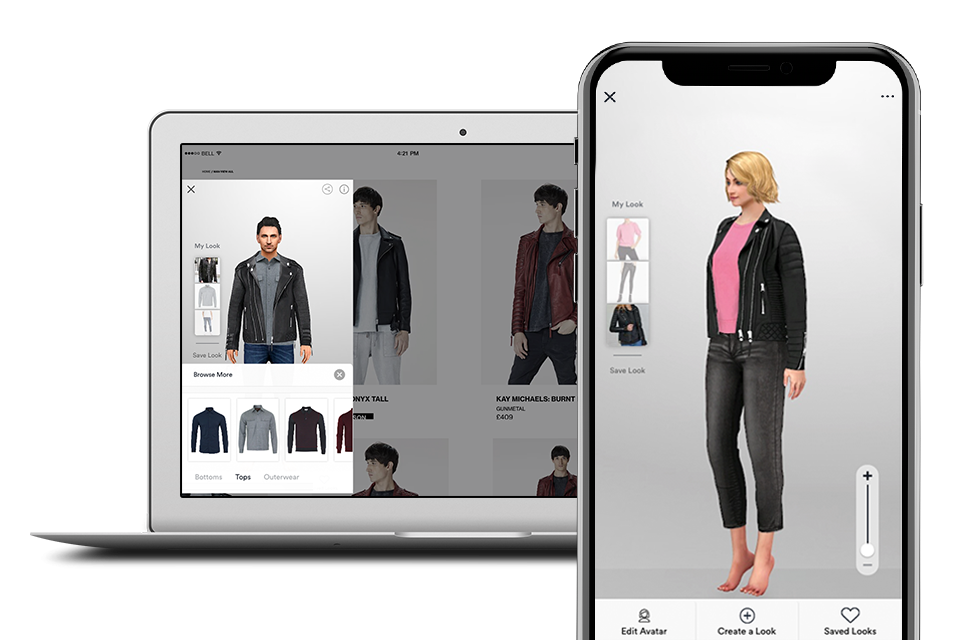The image features a laptop on the left and a cell phone on the right, both with their screens illuminated. The cell phone screen displays a cartoonish avatar of a woman with short blonde hair, standing barefoot, wearing a black jacket, black jeans, and a pink shirt. She appears on her tiptoes, facing left, with options for customization such as "edit avatar," "create a look," and "save look" visible at the bottom. Various smaller images of her in different outfits are shown on the left side of the screen.

The laptop screen also displays an avatar, this time of a man, suggesting the use of the same app for designing avatars. The man is seen on the left side of the screen, wearing a brown denim jacket over a blue shirt. Below him, different color options for the jacket, like brown, light blue, and black, are available. The interface includes sections for "tops," "bottoms," and "outerwear," with "tops" currently selected. Above the man's avatar, more avatars showcasing different jackets are presented. The background of both screens features gray tones, tying the elements together. Both devices are silver-gray, contributing to the cohesive aesthetic of the scene.